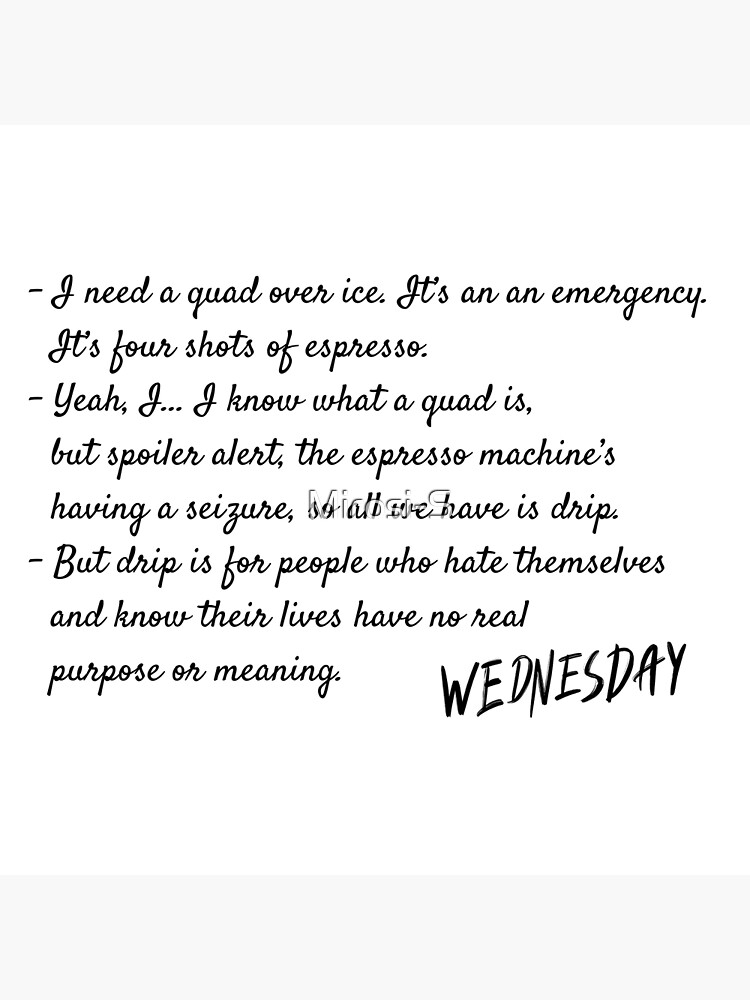The image features black cursive text set against a white background with light gray accents at the top and bottom. The main text reads, "I need a quad over ice, it's an emergency, it's four shots of espresso. Yeah, I know what a quad is, but spoiler alert, the espresso machine's having a seizure. All we have is drip, but drip is for people who hate themselves and know their lives have no real purpose or meaning." On the bottom right, in a different, larger uppercase font, the word "Wednesday" is prominently displayed. Additionally, there is slightly transparent, unreadable text in the center, resembling a watermark that mentions "Mikosa" or "Mikosi S."